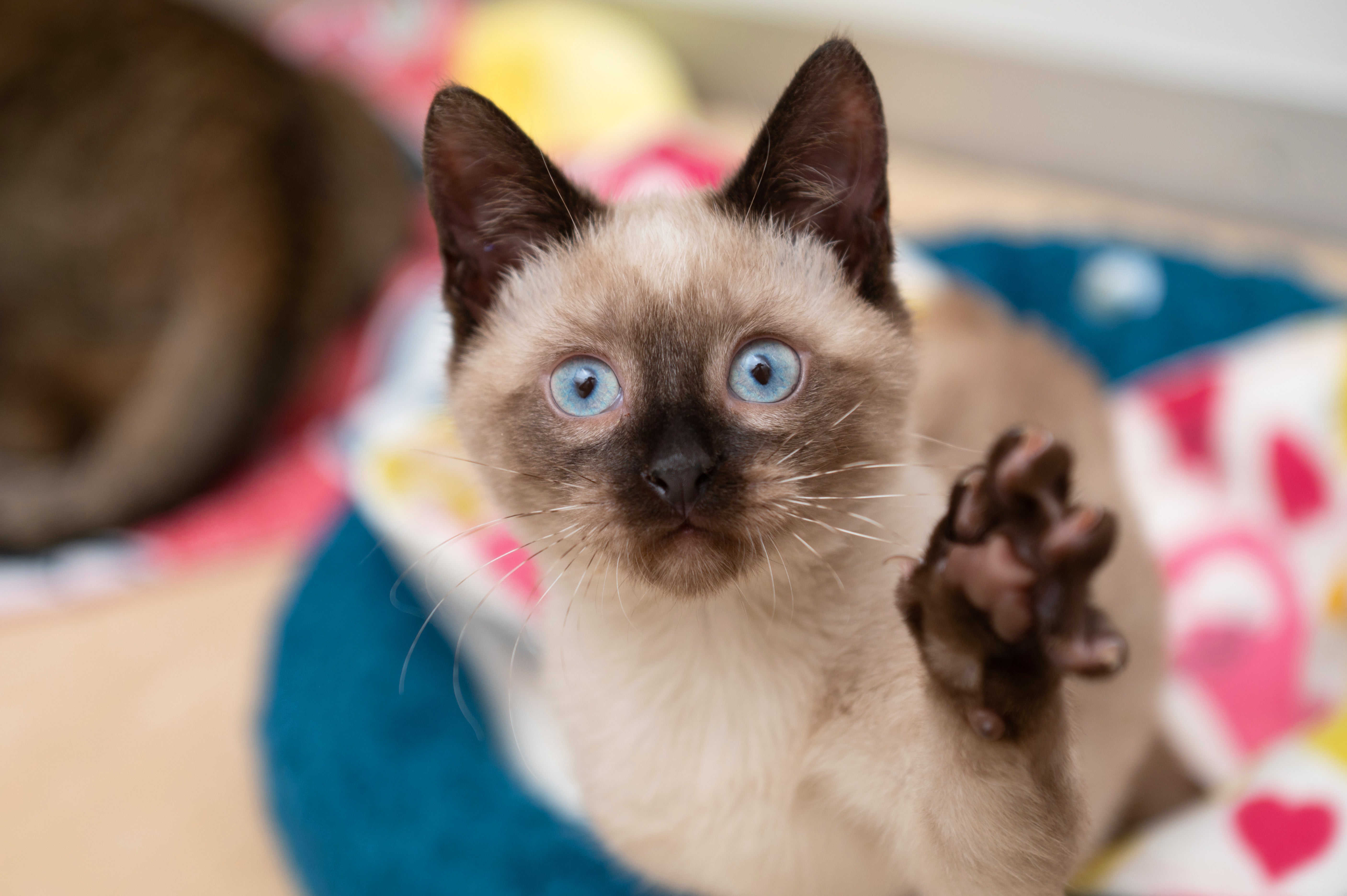This professionally shot image captures a curious Siamese kitten with striking features. Its cream-colored body is accentuated by black markings on its nose, ears, and paws. The kitten, with its beautiful wide blue eyes and long white whiskers, is sitting on a blue, white, and pink blanket. One paw is extended towards the camera, fully displaying its toes and claws. The background, blurred with a strong depth of field effect, reveals the presence of another cat softly out of focus and the tail of a chocolate lab near the edge, adding to the scene's detail and warmth. The setting appears to be a cozy space with a tan floor and various cat beds, including the blue one on which the kitten rests. The captivating and adorable expression of the Siamese kitten suggests its curiosity about the photographer.